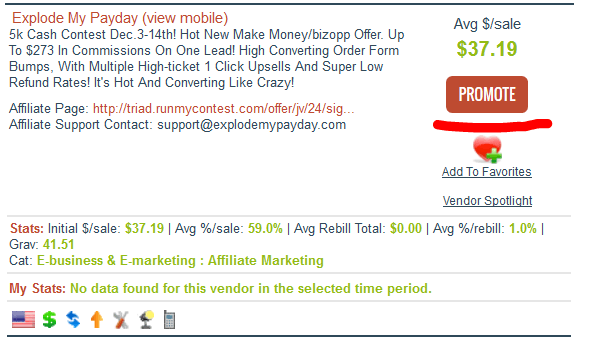This promotional image effectively markets a lucrative opportunity, emphasizing the substantial earnings potential and profitability. 

In the top left corner, bold red text reads "Explode My Payday" with an accompanying note in parentheses, "View Mobile." Below this, more red text announces a "5k Cash Contest" running from December 3rd to the 14th. It highlights a new "Make Money/BizOp" offer, emphasizing the potential to earn up to $273 in commissions from a single lead. 

The image further elaborates on the high conversion rates, mentioning that the order forms feature bumps with multiple high-ticket, one-click upsells, combined with super low refund rates, making this offer exceptionally attractive and profitable.

There is a noticeable gap, and below it, the text guides viewers to the affiliate page, followed by a web address. Further down, it mentions "Affiliate Support Contact" with an accompanying email address, likely to be explode@mypayday.com.

To the right of the image, it states the average money per sale, written as "$37.19." Lastly, there is a prominent red "Promote" button with white text, inviting affiliates to start promoting this high-converting offer.